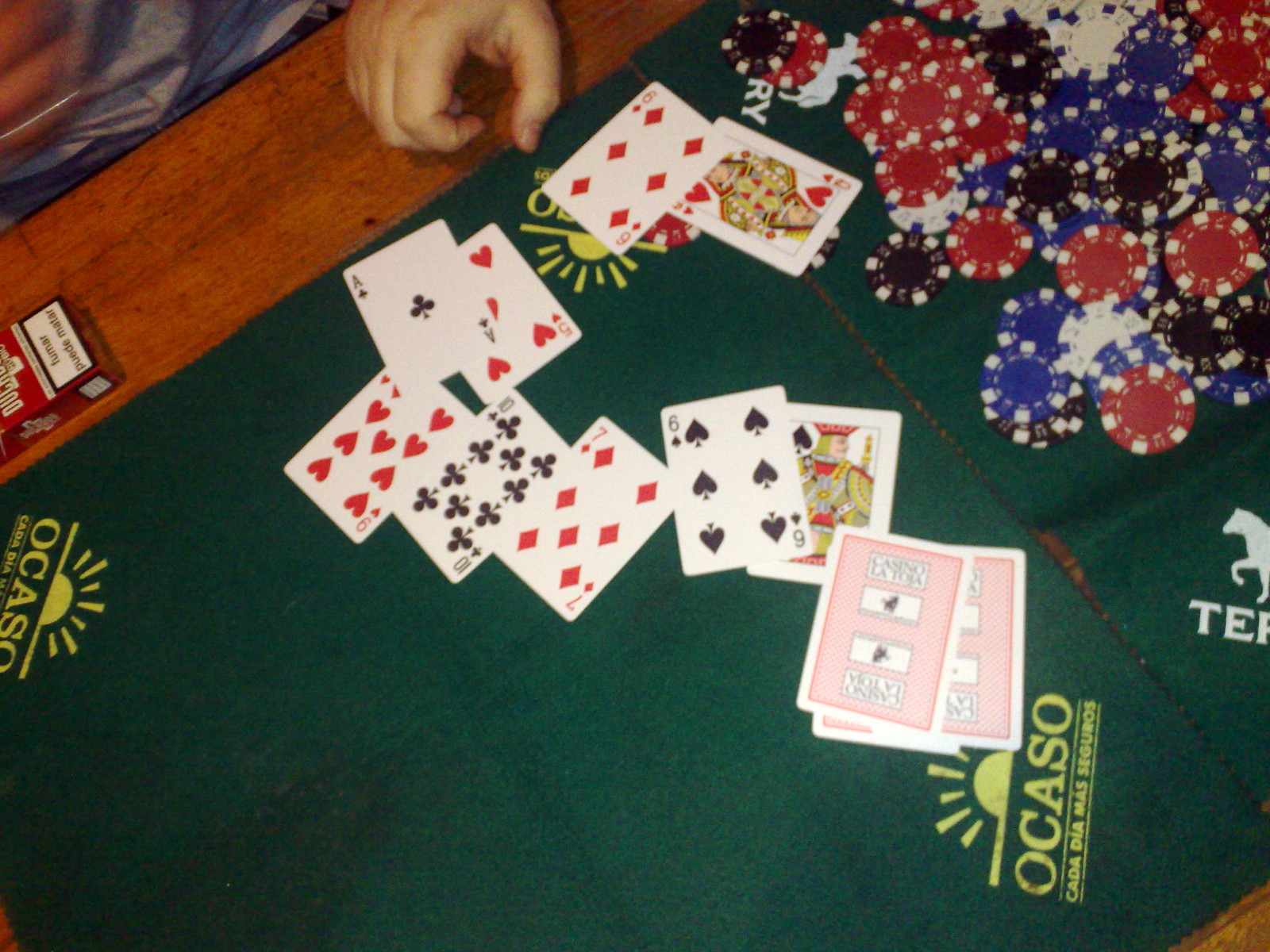The image depicts a vibrant casino table adorned with elegant mahogany wood along its sides. At the center of the table is a green felt surface prominently displaying the company logo "Okaso Karadia Más Seguros," likely the name of the casino. In the upper left of the image, a cigarette box is visible, featuring the health warning "Fumar Puede Matar" (Smoking Kills). 

Scattered across the table are various playing cards: the Ace of Clubs, Nine of Hearts, Five of Hearts, Six of Diamonds, Queen of Hearts, Seven of Diamonds, Ten of Clubs, Six of Clubs, and the King of Clubs. Three additional cards lie face down, their identities unknown. 

Casino chips in black, red, white, and blue hues are situated in the upper-right corner. A partially obscured, faint image of what seems to be a horse or a wolf, accompanied by the letters "T.E.R.," occupies a spot on the table. 

In the upper left-hand portion of the image, the hand of a person appears poised to pick up a card, adding a dynamic element to this detailed casino scene.